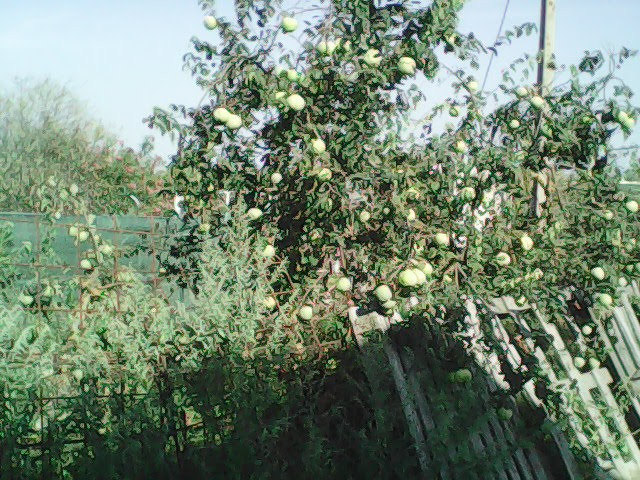This color photograph captures a backyard scene dominated by a large, overgrown green apple tree laden with approximately 40 to 50 green apples. The tree's branches, which appear unruly and uncared for, occupy about two-thirds of the frame. Flanking the apple tree on the left is a variety of shrubbery, while in the foreground an off-white, slightly dilapidated picket fence leans precariously into the tree. Adjacent to this is a section of metal grid fencing. The lush greenery extends into the background where there is more shrubbery and grassy areas, leading to a light gray-blue, cloudless sky, indicating a sunny day. Scattered white flowers are also visible among the greenery, adding to the wild, untended look of the scene.